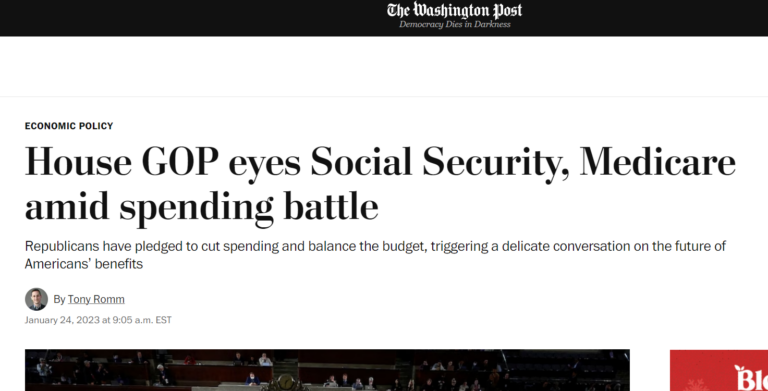The image depicts a section of the Washington Post website. At the top of the page, there's a black banner with the phrase "Democracy Dies in Darkness" written in white. Below this banner, the Washington Post logo is prominently displayed, also in white. The headline underneath reads, "Economic Policy: House GOP Eyes Social Security, Medicare Amid Spending Battles." The article provides an in-depth analysis of the Republican party's intentions to cut spending and balance the budget, igniting a nuanced conversation on the future of American benefits. The article is authored by Tom Romm and is dated January 24th, 2023, at 9:05 a.m. EST.

The page also features a narrow, dark horizontal image of the U.S. Congress, specifically the House of Representatives. At the bottom right of this image, there is a blue rectangle with partially visible white text that starts with "BL," but the rest of the text is cut off and indecipherable. The overall color scheme of the webpage predominantly features black, white, and red. The most striking text is the headline concerning the House GOP's focus on Social Security and Medicare during spending battles. The photo is notably dark, making it difficult to discern specific colors and details within the image.